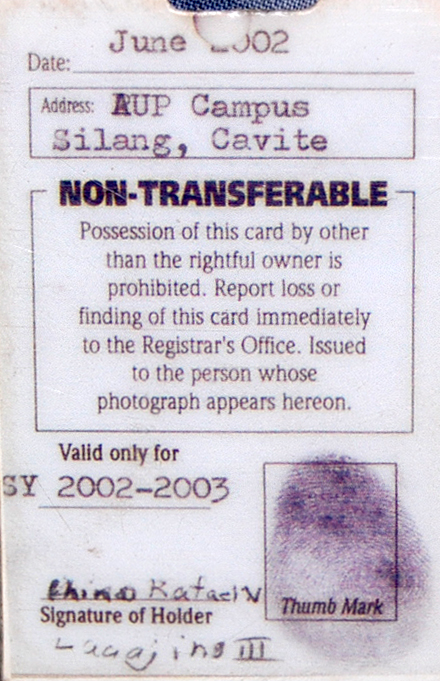The image exclusively features a single object, which is a close-up of a card that occupies the entire frame. This well-worn card, likely issued by a campus, bears several important details. At the top, it prominently displays the date, June 2002. The card provides the address "AUP Campus Silyang Cavite" and includes a strict notice stating, "Non-transferable. Possession of this card by other than the rightful owner is prohibited." It also instructs to "Report loss or finding of this card immediately to the registrar's office." Further details specify it was issued to the individual whose photograph appears on it and is valid only for the school year 2002-2003. There is a designated space for a thumb mark, which bears an inked fingerprint, and another for the signature of the holder. The colors on the card include shades of white, black, gray, purple, and blue, indicating its aged and possibly rough condition. Handwritten elements on the card include names that resemble "Rhino Raphael" and "Lui Jing 3."